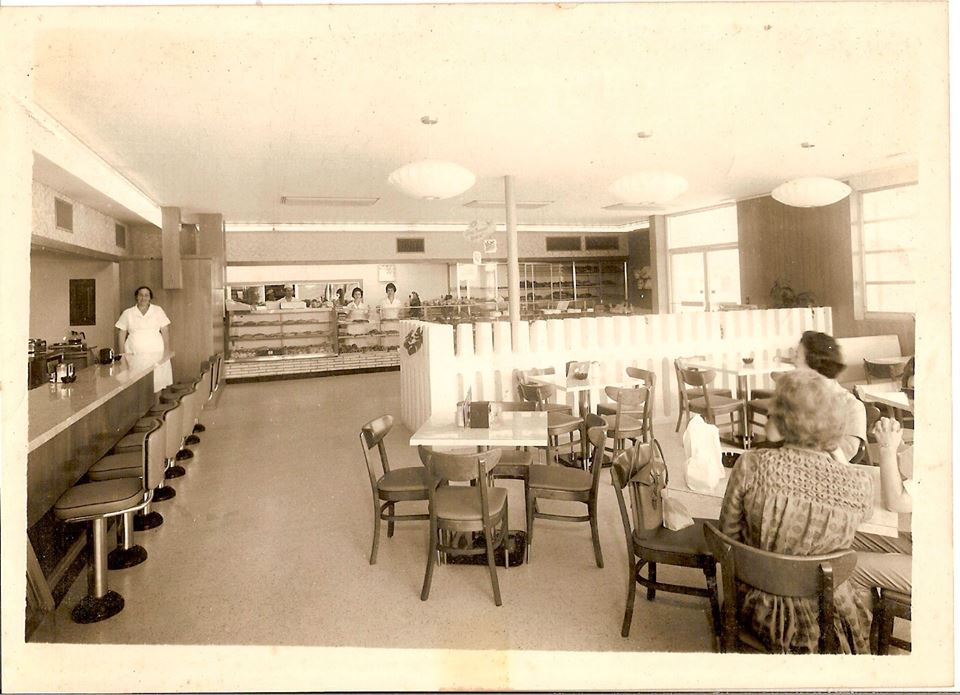The black and white photograph, likely from the 1950s, captures a quintessential mid-20th-century diner. This restaurant, possibly doubling as a bakery, features a decoratively quaint white picket fence that partitions off certain areas. The floor glistens with a laminate finish, and standard square white tables with four chairs each are arranged throughout the room. Two women are seated at one of these tables, engaging in conversation against the nostalgic backdrop.

To the left, a bar area is visible with several stools lined up in front of it, while on the right, a dining area extends, separated by the noted white divider. In the background, the counter is staffed by women dressed in white short-sleeved shirts and knee-length flowing skirts typical of the era's service attire. At the far end near the counter, various pastries and food items are on display.

Besides the two customers, three women—the staff—are also captured in this scene. One waitress stands by the coffee pots in a corner, while the other two seem engaged near the back, possibly conversing about their duties. A hint of another worker can be noticed, slightly cropped off the right edge of the photograph. The overall setting epitomizes the serene yet industrious atmosphere of a classic 1950s diner.